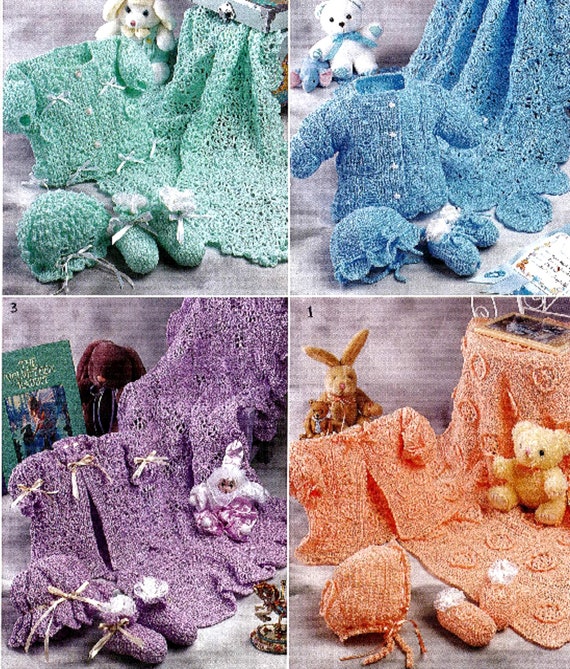This image features a collage of four photographs, each showcasing a set of colorful knitted baby outfits accompanied by matching blankets and stuffed animals. In the top left corner, labeled with the number one, there is a teal baby ensemble including a shirt, cap, shoes, and a bunny dressed in teal. Adjacent to it in the top right corner is a blue set consisting of a shirt with white buttons, bonnet, shoes with white interiors, and a white bear with a blue bow tie. The bottom left photograph, labeled with the number three, displays a purple set with a dress, bonnet, shoes, and a brown stuffed bunny. Finally, the bottom right corner features a pinkish-coral outfit labeled number one again, with a blouse, bonnet, shoes, and both a stuffed rabbit and a teddy bear. Each set is meticulously presented in separate boxes but unified in the collage, highlighting their knitted craftsmanship and vibrant colors.